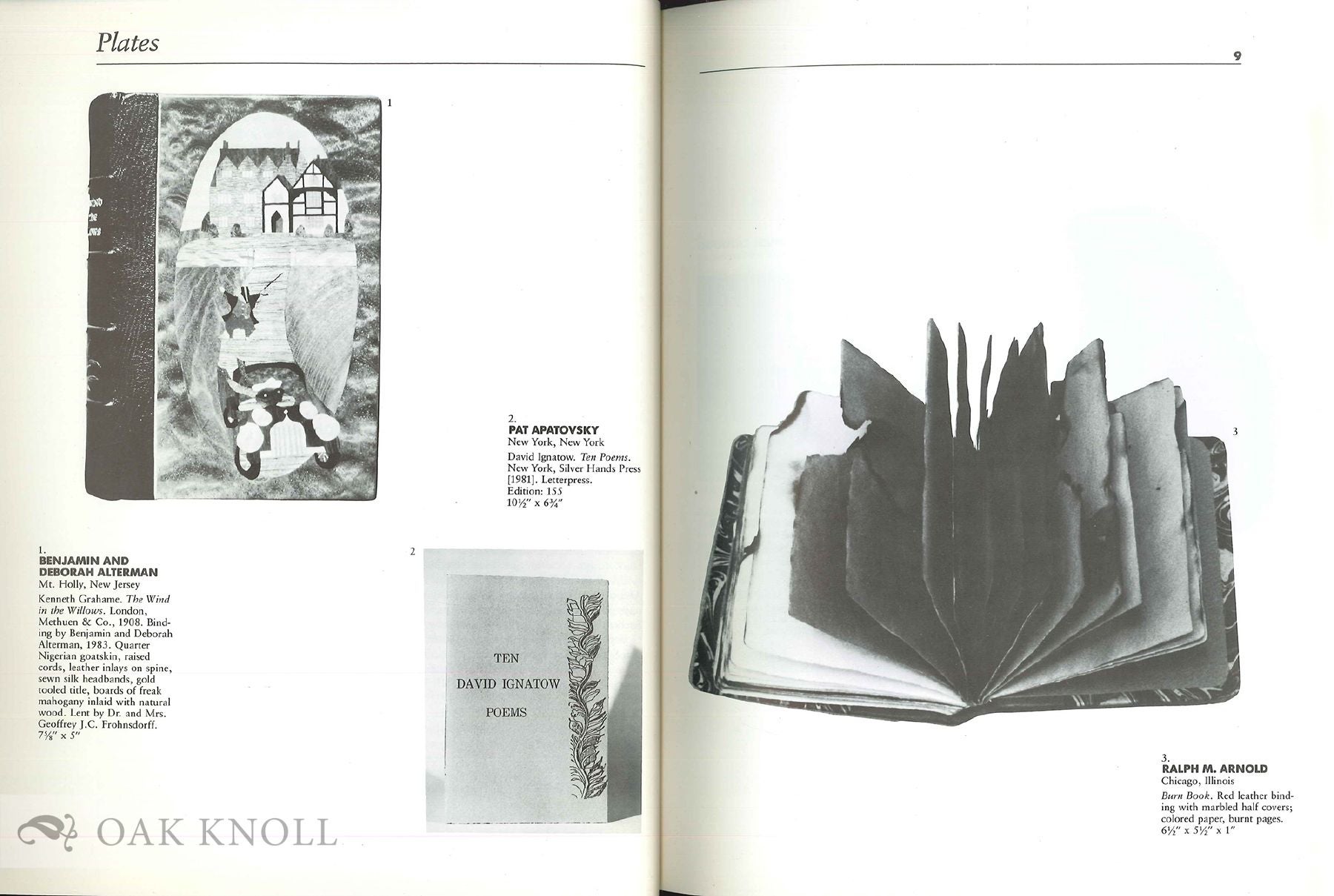The image depicts an opened booklet, displayed in black and white, showcasing detailed descriptions of three distinct books. On the top of the left page, the word "Plates" is elegantly italicized. Below this, a photograph captures "The Wind in the Willows" by Benjamin and Deborah Alterman from Mount Holly, New Jersey, dated 1908. This image features a fantasy house, with a man in a top hat, vest, and jacket, holding a cane beside a character in a convertible car. Adjacent to this, is the second book titled "10 David Ignatow Poems" by Pat Epitofsky from New York.

The right page presents a striking image of a distressed and raggedy book by Ralph M. Arnold from Chicago, Illinois. The book, bound in red leather with marbled half covers, exhibits burnt edges and torn pages, reflecting significant age and wear, and includes colored papers. The dimensions of this book are noted as six and a half inches by five and a half inches by one inch. The descriptions and the photographs are finely printed in black and white providing a rich, visual catalog of these unique and historically significant items.